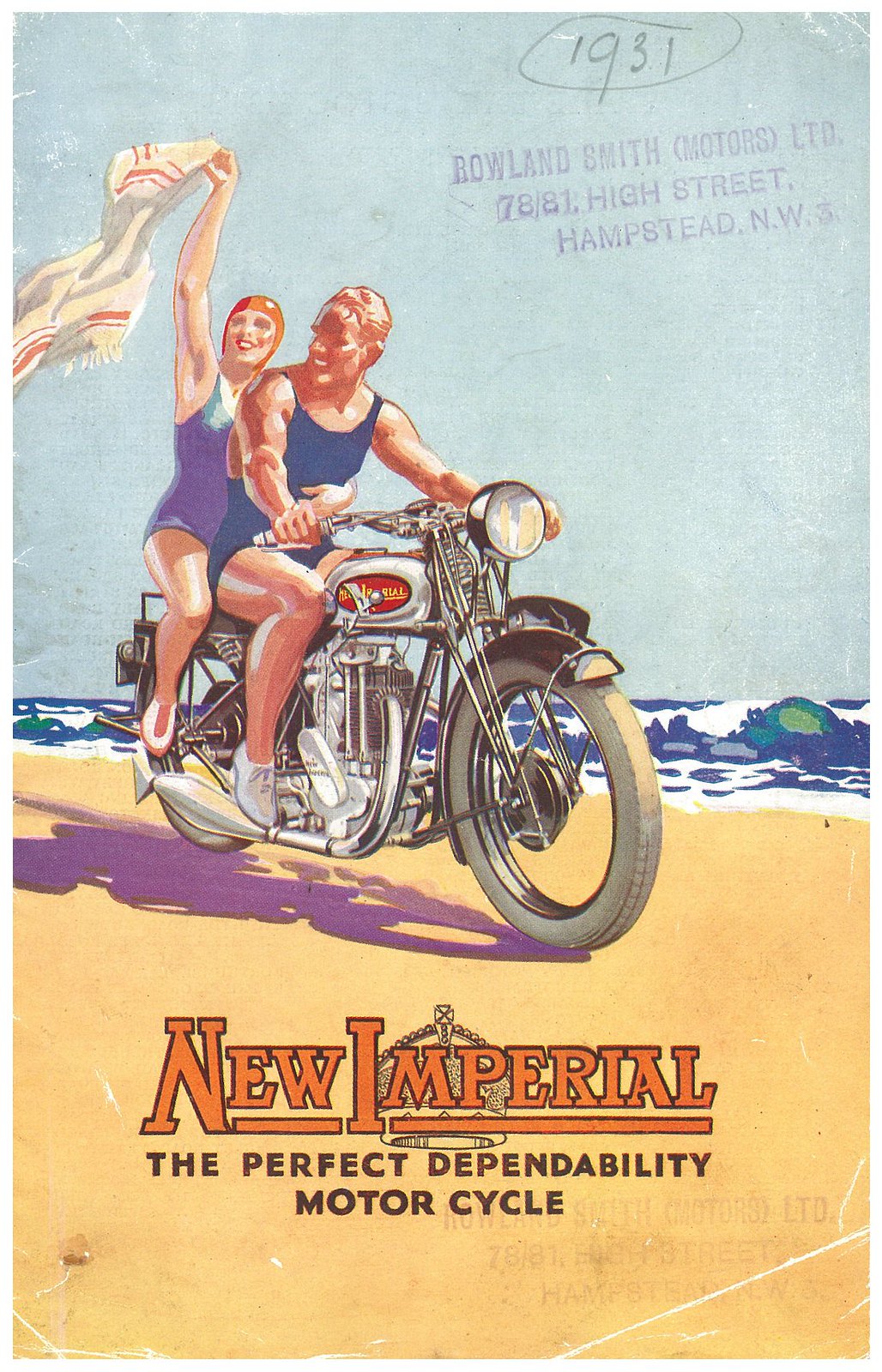This vintage advertisement, styled in Art Deco, showcases a man and woman riding a silver motorcycle adorned with a red logo along a sandy beach. The scene is set against a backdrop of the shoreline and blue, white-capped waves, beneath an open sky. The man is clad in a blue short unitard, while the woman sports a blue bathing suit along with a matching swimming cap and holds a towel aloft. The sand beneath the motorcycle bears the bold orange inscription "New Imperial," followed by "The Perfect Dependability Motorcycle" in black. In the upper right corner, a penciled "1931" is circled, with a blue stamp below it reading "Roland Smith Motors LTD, 7881 High Street, Hampstead NW3." This stamp appears again, albeit faintly, in the bottom right corner. Visible distress marks such as scratches and folds hint that this image is a scanned copy of the original ad.